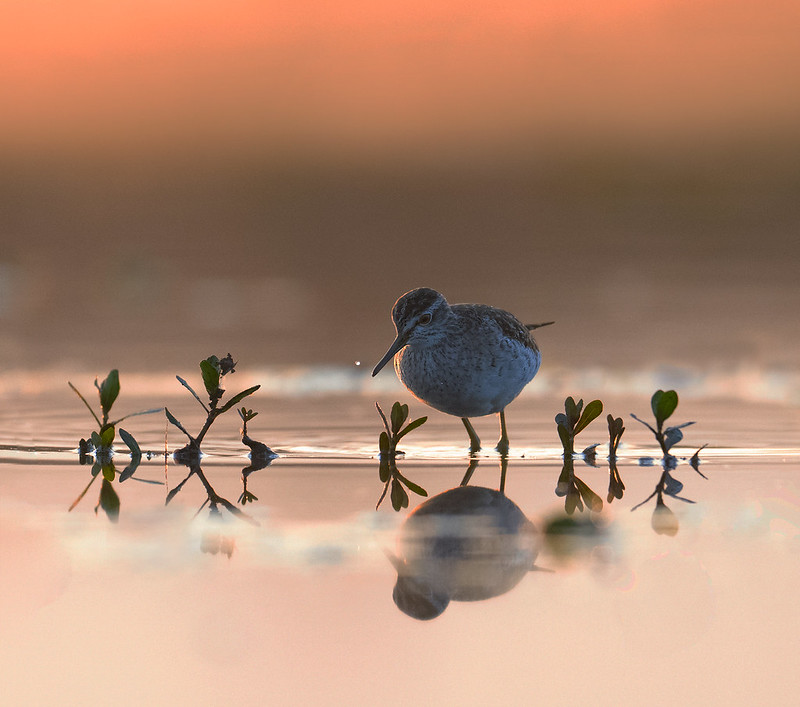The photograph captures a small bird standing in shallow water, with half of its legs submerged. The bird has a long beak and is adorned with white and brown feathers. Around the bird, there are small plants emerging from the water, their green leaves and budding petals visible. The water acts like a mirror, reflecting both the bird and the plants. The background suggests either sunrise or sunset, with blurred warm hues of orange, beige, and pink, adding to the tranquil ambiance. The smooth water surface hints at the gentle waves nearby, and the overall scene is serene and picturesque, portraying the beauty of nature in a calm, reflective moment.